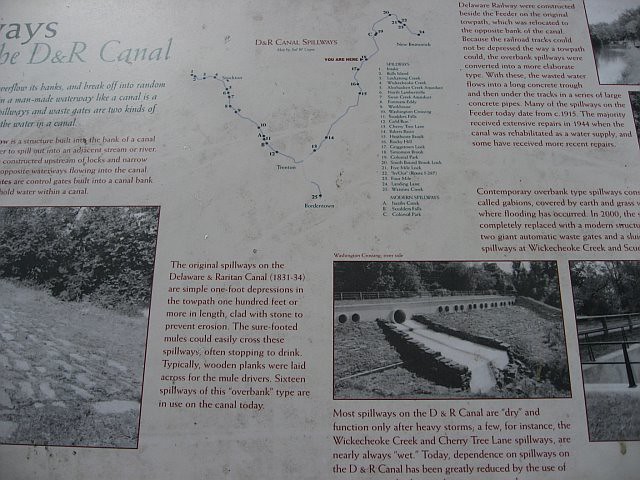This photograph captures a detailed bulletin board or scrapbook-like display, prominently featuring a collection of black-and-white photos. Each photo is accompanied by descriptive text, providing context and information. The central theme appears to be the DNR Canal, as indicated by a partially visible placard. Among the photographs, one in the center seems to depict water being directed through an aqueduct, highlighting an aspect of the canal's function. A meticulously drawn map is also part of the display, annotated with a lengthy list of approximately 15 locations, likely tracing the canal's route. The display is crowded with text, arranged in several columns, though some of this text is difficult to read due to the partial view. The overall impression is of a densely informative and visually engaging documentation of the canal and its associated sites.